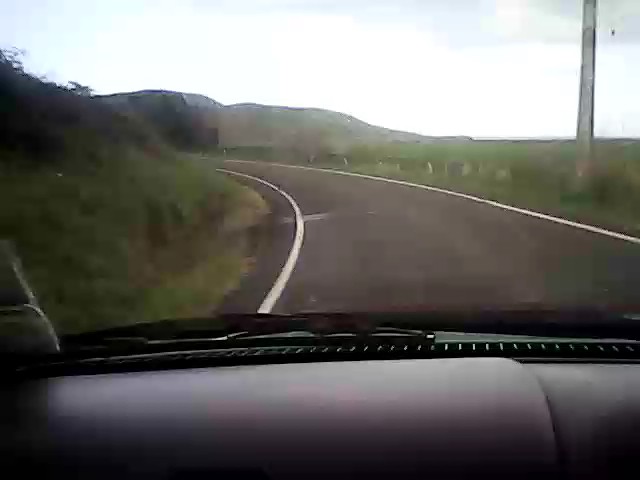This low-quality, pixelated color photograph appears to be taken from the inside of a car, likely from the passenger side, suggesting a right-hand drive vehicle typical of regions like Europe or the UK. The foreground of the image prominently features the car's dashboard and the base of the windshield wiper. Through the windshield, we can see a long stretch of highway, with white lines demarcating either side of the road. The road curves gently to the left, bordered by green grassy expanses that extend towards a backdrop of large hills or a mountain range. There are patches of brush visible to the left side of the dashboard. In the top right corner of the image, there is a vertical object, likely a large electrical pole or telephone pole. Above, the sky is a mix of blue with some dark clouds, adding to the overall blurry and textured feel of the photograph.